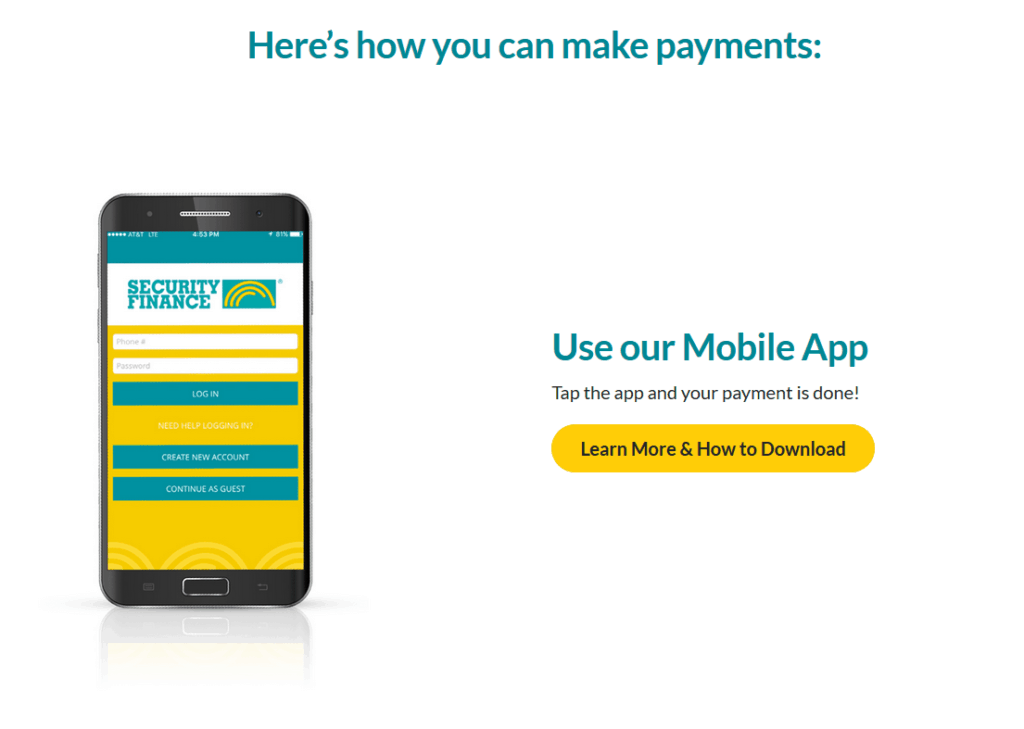This screenshot depicts a web page designed to facilitate mobile payments. The design features a predominantly white background without a border, emphasizing clarity and focus on the content. 

At the top of the image, bold text in an aqua or teal font reads: "Here's how you can make payments." 

On the left side, there is a detailed illustration of a smartphone with a black border and a finely rendered shadow underneath. The screen of the illustrated phone displays a sleek interface primarily composed of white, yellow, and teal colors. Prominently shown is the "Security Finance" title along with its logo, in corresponding yellow and teal hues. This interface includes two input fields for a phone number and password, alongside three blue buttons labeled "Login," "Create New Account," and "Continue as Guest." The phone's screen background features yellow accents with semicircle designs at the bottom, adding a touch of modern aesthetic. The phone itself includes a functional button at the bottom.

To the right side of the illustration, bold teal text declares, "Use our mobile app." Below this, a subheading in the same teal font reads: "Tap the app and your payment is done." A large yellow oval-shaped button, set against a yellow background and accompanied by directional text, prompts users to "Learn more and how to download." 

This detailed and visually appealing layout effectively guides users through the process of making mobile payments using the application.